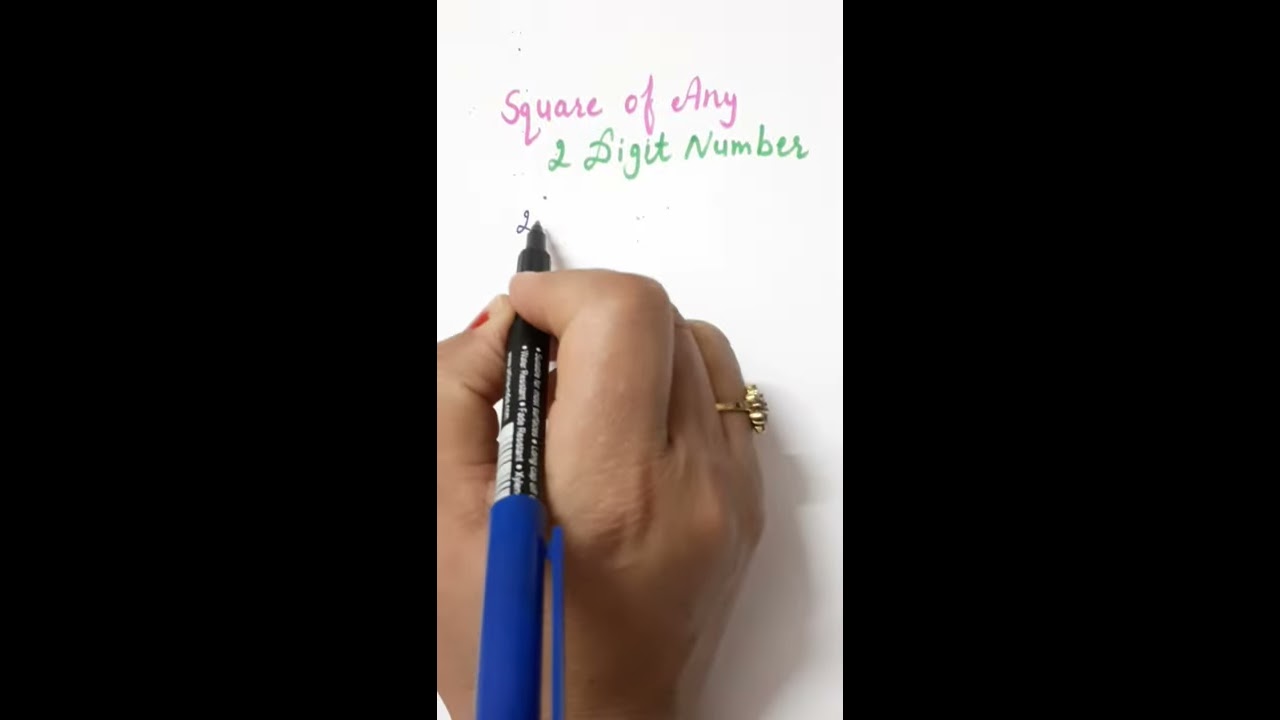The image depicts a color photograph of the top of a woman's hand with olive skin, poised to write on a piece of white paper. Her right hand holds a fine-tipped black pen with white writing and a blue cap. On her right ring finger, she wears a gold ring. There is a hint of red nail polish on her thumb, but the other fingernails are not visible. The writing on the paper, in cursive and multicolored ink, starts at the top with "square of any" in pink, followed by "two digit number" in green, where the number two is a digit. Beneath that, the pen is poised to continue writing, with the cursive letter "L" already visible in black ink. The photograph is long and narrow, flanked by black rectangles on either side.